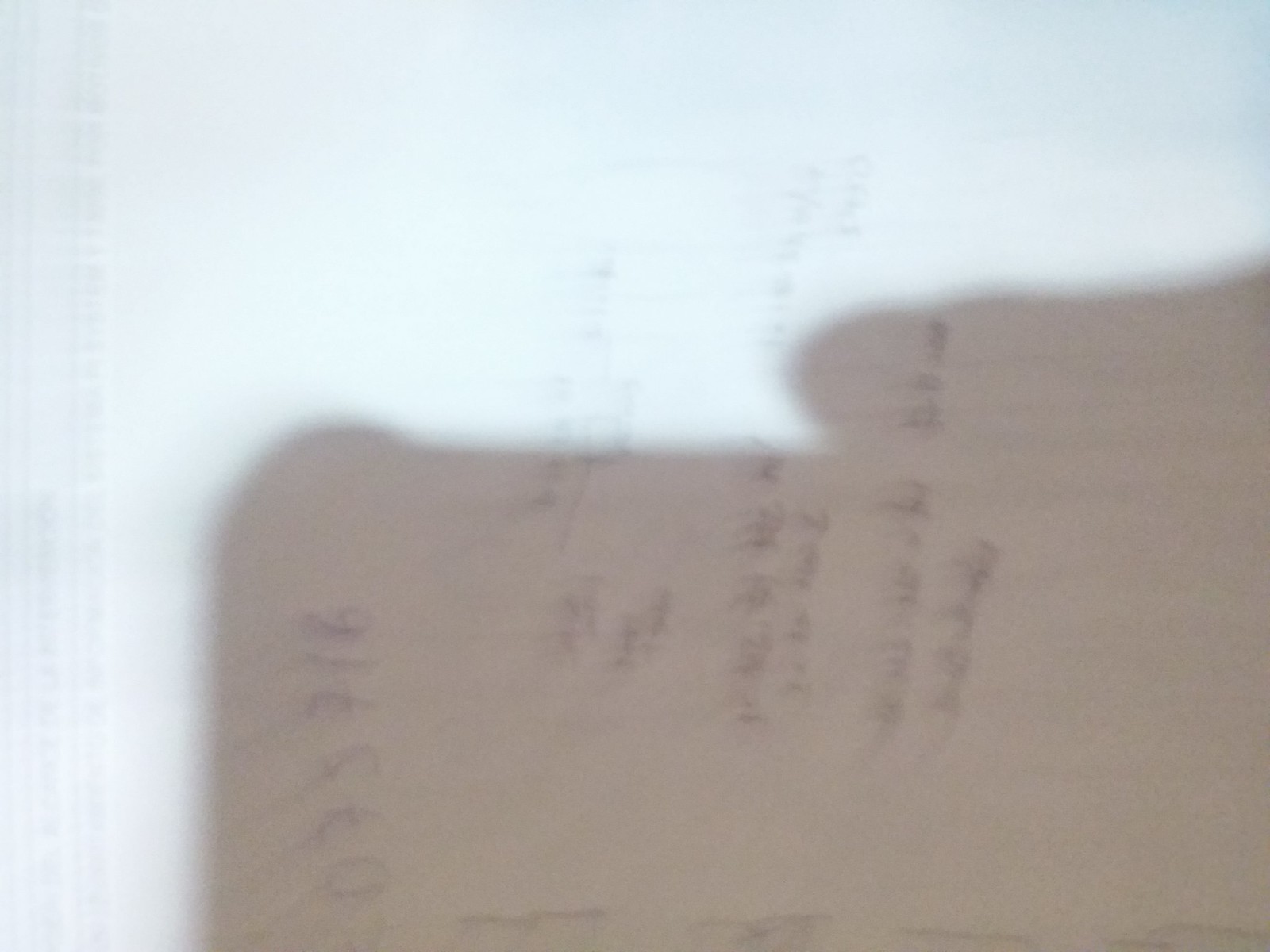In this image, a sheet of paper is shown with very faintly scribbled writing, almost illegible. A shadow dominates the bottom portion of the picture, revealing a hand holding a phone, presumably capturing the snapshot. The shadow extends from the bottom right, covering roughly half of the image. Orienting the image sideways, one can discern fragments of the writing, including scattered numbers such as "07S" and "716," along with a few faint, pencil-written sentences. Additionally, hints of more information appear to bleed through from the other side of the paper, adding to the complexity and obscurity of the text.